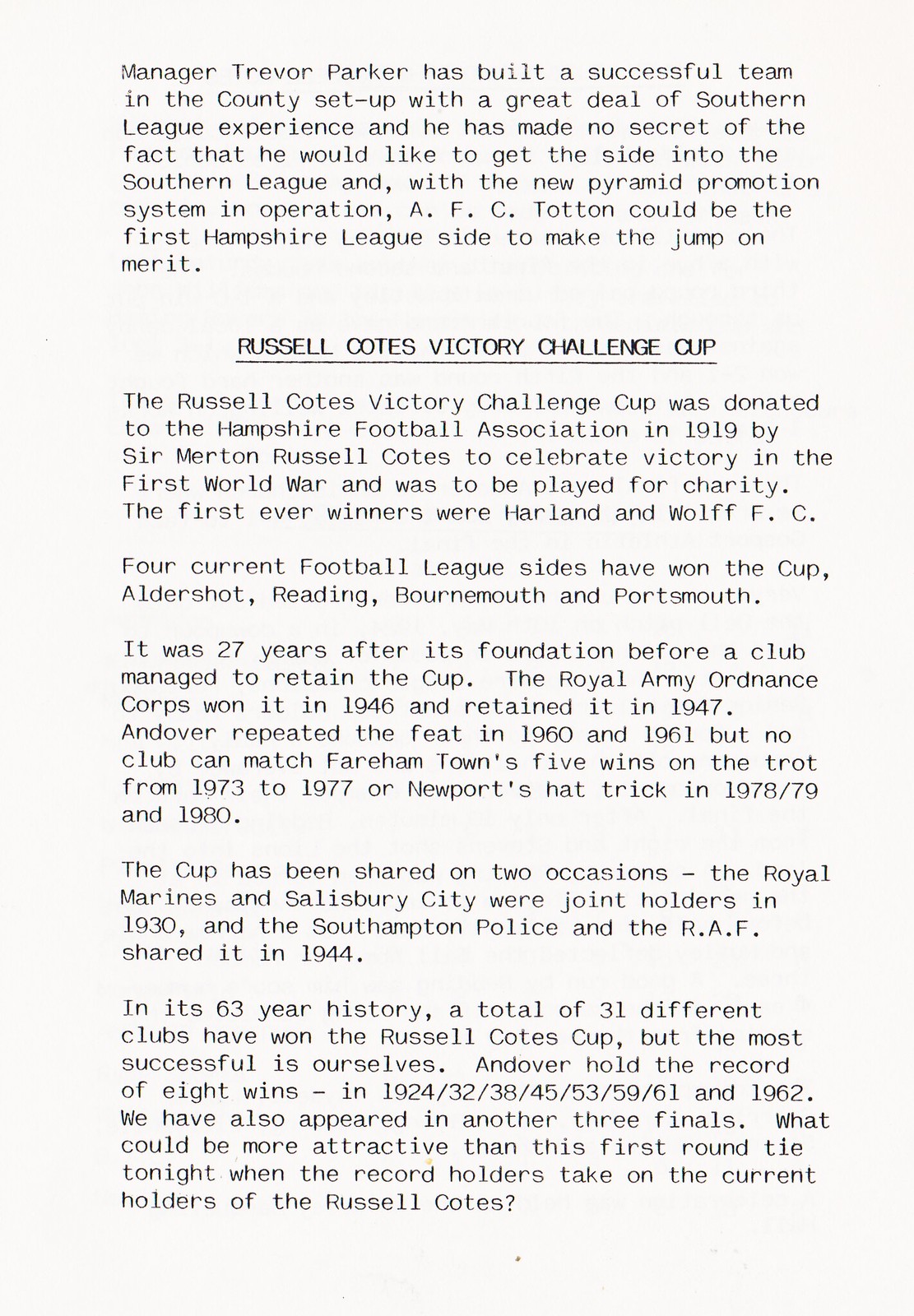The scanned image displays a piece of paper with black font printed on a white background. At the top, it features a paragraph highlighting Manager Trevor Parker's efforts in building a successful team in the county. It emphasizes his ambition to advance the team into the Southern League, noting that AFC Totton could be the first Hampshire League side to achieve this through the new pyramid promotion system. Below this paragraph, the heading "RUSSELL COATES VICTORY CHALLENGE CUP" is prominently bolded and underlined. The text goes on to explain that the Russell Coates Victory Challenge Cup was donated to the Hampshire Football Association in 1919 by Sir Merton Russell Coates to commemorate victory in the First World War and was intended to be played for charity. It details the first winners, Harland and Wolff F.C., and notes that four current football league sides—Aldershot, Reading, Bournemouth, and Portsmouth—have won the cup. The narrative further elaborates on the cup's history, mentioning notable achievements such as the Royal Army Ordnance Corps' consecutive wins in 1946 and 1947, Andover's repeated victories in 1960 and 1961, Fareham Town's five straight wins from 1973 to 1977, and Newport's hat trick from 1978 to 1980. The remaining two paragraphs at the bottom continue to describe the historical significance and accomplishments related to the cup and the team.